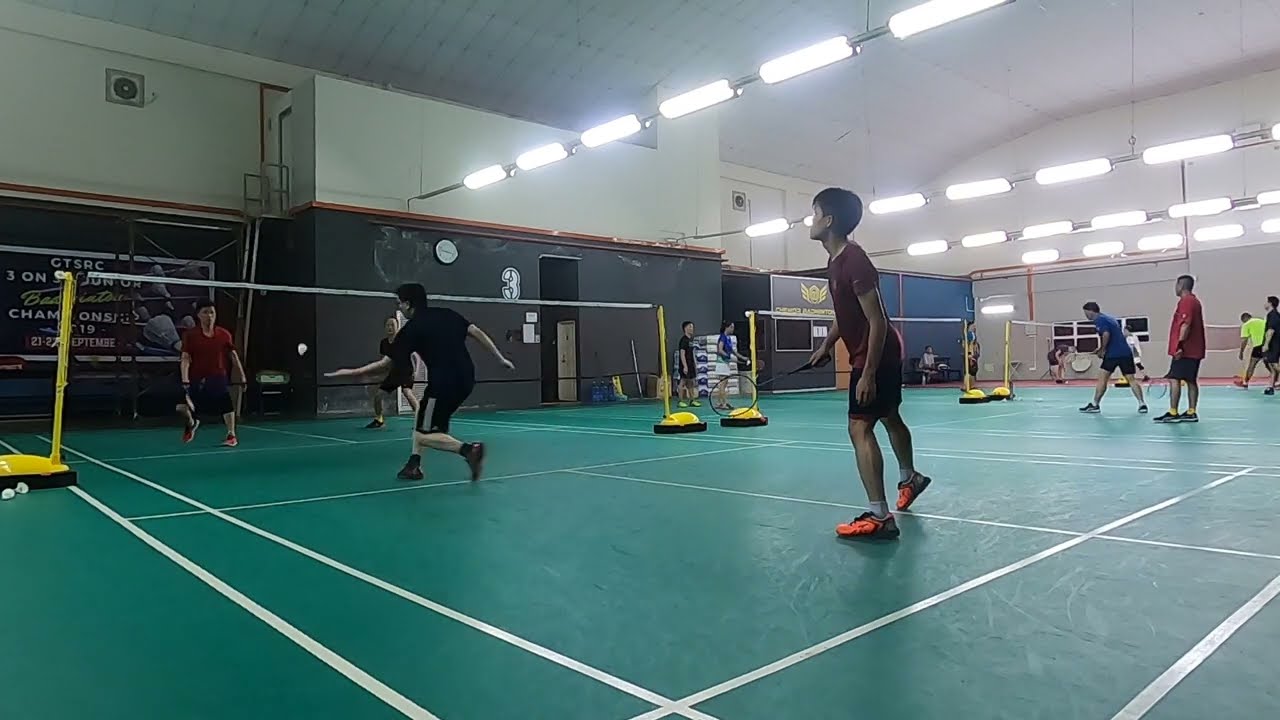The image captures an indoor gymnasium specifically designed for badminton games. The gym features three active badminton courts, each outlined with white markings against a green floor. The walls, both far right and to the side, are painted gray, while the ceiling above is white, showcasing rows of fluorescent lighting. Ventilation units are visible atop the first court. Each court is occupied by male players engaged in doubles matches. On the first court, the player nearest to the viewer sports a maroon short-sleeved t-shirt, black shorts, and neon orange shoes. His teammate, dressed in a black shirt and trousers, is hitting the shuttlecock with his left hand. In the background, players on the second court are preparing for a serve, while on the third court, a player moves to pick up a fallen shuttle. The badminton nets, held by yellow stands, are set low across the courts, and multiple white shuttlecocks are seen in play under the bright, evenly distributed lighting.